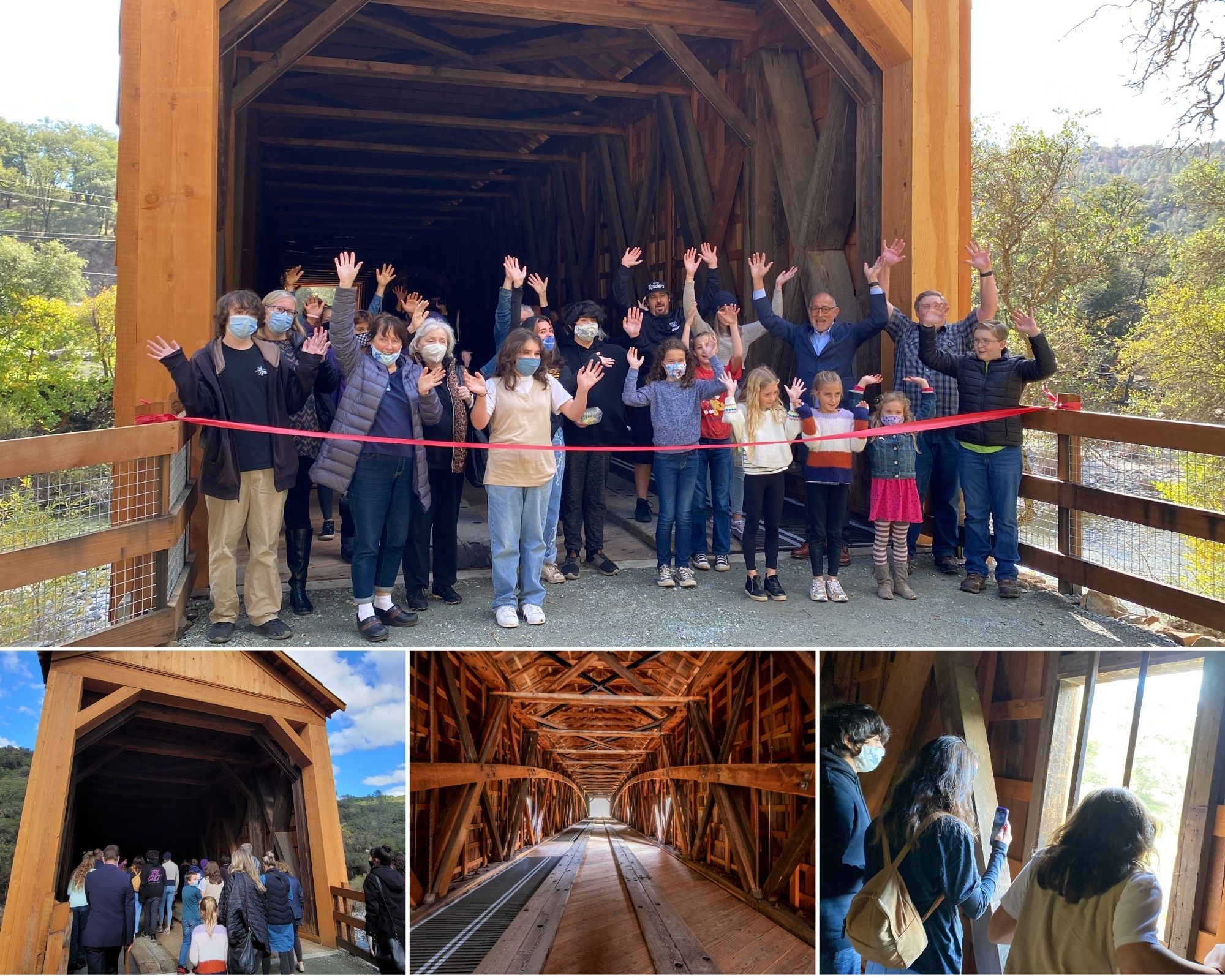Four photographs depict various angles of a wooden tunnel situated in a natural area filled with trees and a river flowing underneath. The top photograph shows a ribbon-cutting ceremony at the tunnel’s entrance, featuring a large group of people of various ages, some wearing masks, all with raised hands in celebration behind a big red ribbon. The bottom left image displays these people from the back as they walk into the tunnel. The bottom center photo provides a detailed interior view of the tunnel, highlighting the complex arrangement of wooden planks. The bottom right photograph captures a few individuals standing inside the tunnel, looking out of a window on the right side, with one person appearing to hold a camera, dressed in a dark long-sleeve shirt and a backpack.